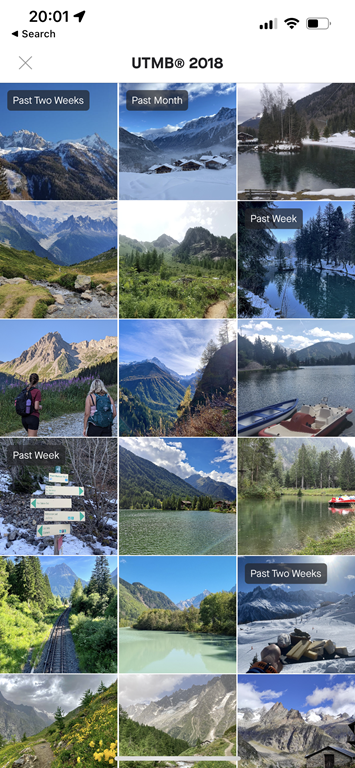The image displays a comprehensive gallery of mountainous landscapes, organized on a white background. Dated 2001, a black arrow points to the upper right corner, adjacent to a left-pointing search button and an 'X' in the center. The text "UTMB ® 2018" is prominently displayed. In the top right corner, icons for signal bars and battery status are visible.

The gallery consists of approximately 18 images, showcasing a variety of high-altitude scenes characterized by snow-capped mountains under a clear blue sky. The gallery is segmented into different timelines: "Past Two Months," "Past Month," and "Past Week," each labeled in black boxes with white text.

For the "Past Two Months" section, the images largely depict snowy mountain peaks with occasional glimpses of lakes and forests, showing less snow at lower elevations.

The "Past Month" section features:
- A snowy mountainous landscape.
- A partially snow-covered lake surrounded by trees and mountains.
- A mix of green foliage with minimal snow in the valleys.

Moving to the "Past Week" section, the gallery includes:
- Snow-laden trees and a lake with a snowy backdrop.
- A vibrant image of mountains under a clear sky with two hikers.
- A clear day with no snow.
- Slightly snowy terrain.
- A road sign with five directions.
- Images of clear vistas, lakes with boats, roads with mountain views, and lush greenery.

Lastly, the "Past Two Weeks" section highlights: 
- A heavily snow-covered scene.
- Green hillsides beneath cloudy skies.
- Green expanses with distant snowy peaks.
- An exceptionally breathtaking landscape.

Each photo vividly captures the dynamic and picturesque nature of the mountainous area across different timescales.